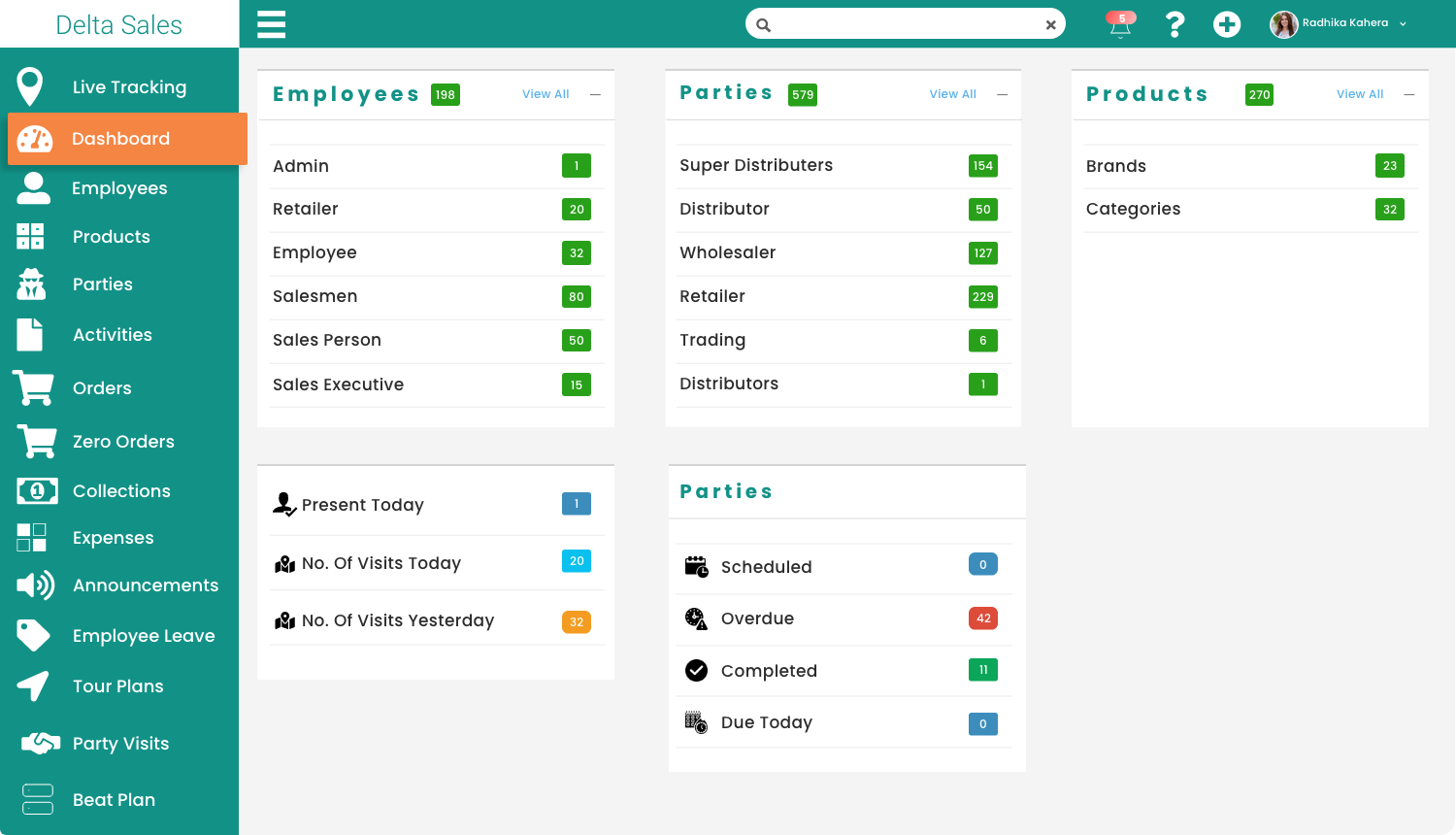The image is a screenshot of the Delta Sails application interface, optimized for a desktop computer with a wider-than-tall aspect ratio. The color scheme features predominantly white, gray, and green-teal hues. In the upper left-hand corner, within a white rectangular section, the text "Delta Sails" appears in a green-teal font.

The top bar of the interface includes several key elements: three horizontal white lines on the left, likely representing a menu; a search bar; and various icons including a notification bell, a question mark, a plus sign, and a circular headshot image accompanied by the name "Radhika Kehera." 

On the left-hand side of the screen, positioned under the "Delta Sails" header, is a vertical menu in green-teal. This menu provides access to various tools and sections such as Live Tracking, Dashboard, Employees, Products, and Beat Plan. The Dashboard option is highlighted by an orange rectangle, indicating the user's current selection.

The main window, set against a gray background, displays five distinct boxes labeled Employees, Parties, Products, Parties, and a detailed sales reporting dashboard. The sales reporting dashboard, located in the lower left of the main window, provides metrics such as "Present Today," "Number of Visits Today," and "Number of Visits Yesterday," offering a snapshot of recent sales activity and performance.